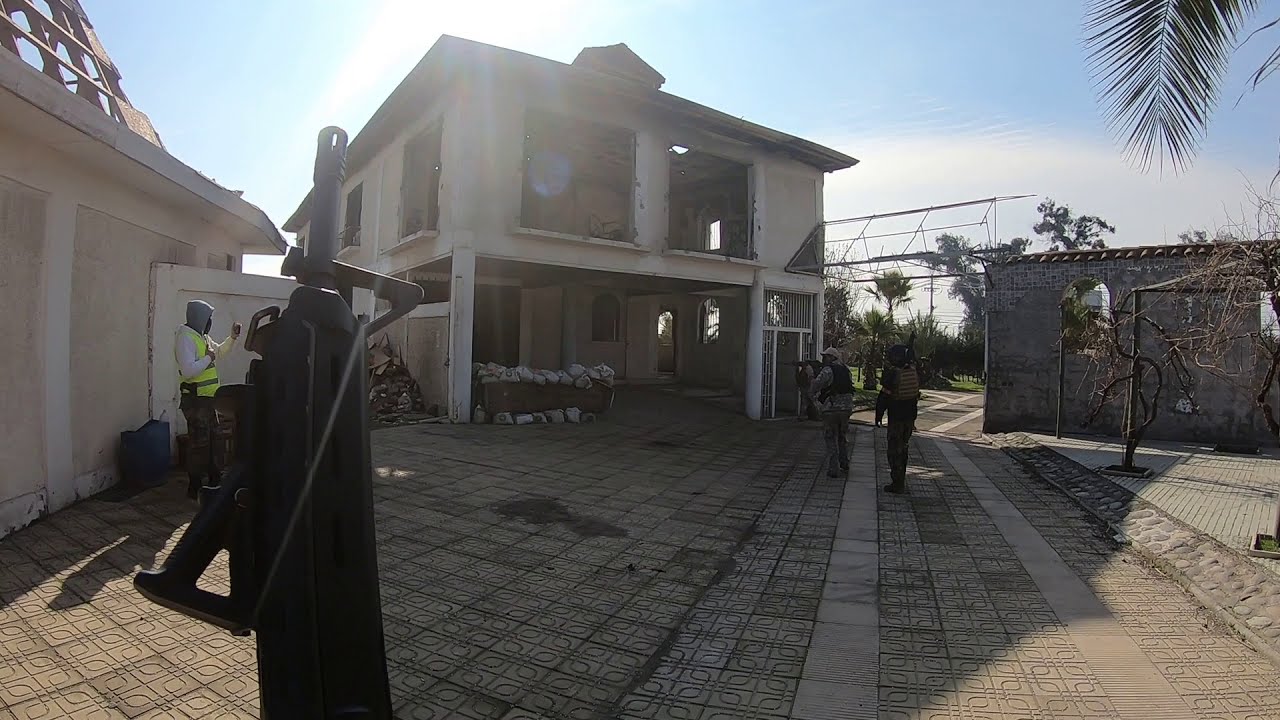This image depicts a rundown, two-story building with blown-out windows, situated in a stone courtyard with distinct spade-design stonework. The scene is set outdoors during the daytime, under a blue sky, with sunlight casting shadows outward from behind the building. Scattered around the courtyard are numerous empty garbage bags and sandbags, adding to the abandoned and deserted atmosphere.

In the courtyard, there are three individuals, all involved in a tense situation. In the foreground, two men wearing military-style gear and bulletproof vests face left, with one pointing a rifle in that direction. To the left, another man, dressed in a yellow safety vest and white long-sleeve shirt with a hoodie, stands with his hands raised. Additionally, a palm tree is visible in the upper right corner of the image. It appears that the photographer, or cameraman, is also holding a gun pointed upwards, emphasizing the intensity and potential conflict in the scene.